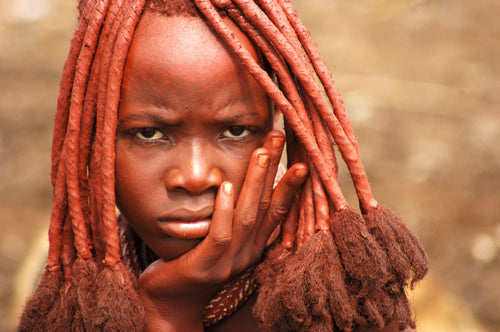In this detailed and evocative portrait, we see a young black woman with a striking and unique hairstyle. Her hair is styled into long, tightly woven braids or dreadlocks that cascade down on either side of her face, resembling orange ropes. The ends of these braids are adorned with brown, tassel-like puffs, adding to the textured look. A red or pinky-orange hue covers her forehead and intricately coats each strand of hair, suggesting a possible cultural or artistic influence. The same red coloring is seen scattered across her face and hands, which she rests thoughtfully on her cheek, with her four fingers nestled against her chin and lower face. Her expression conveys a sense of frustration or contemplation, as her gaze is directed slightly upward and forward. The blurred background, showcasing a brownish, light beige tone, places the focus solely on her, highlighting her expressive features and the vivid details of her appearance. Overall, the image captures the essence of a woman deeply immersed in a moment of introspective stillness.